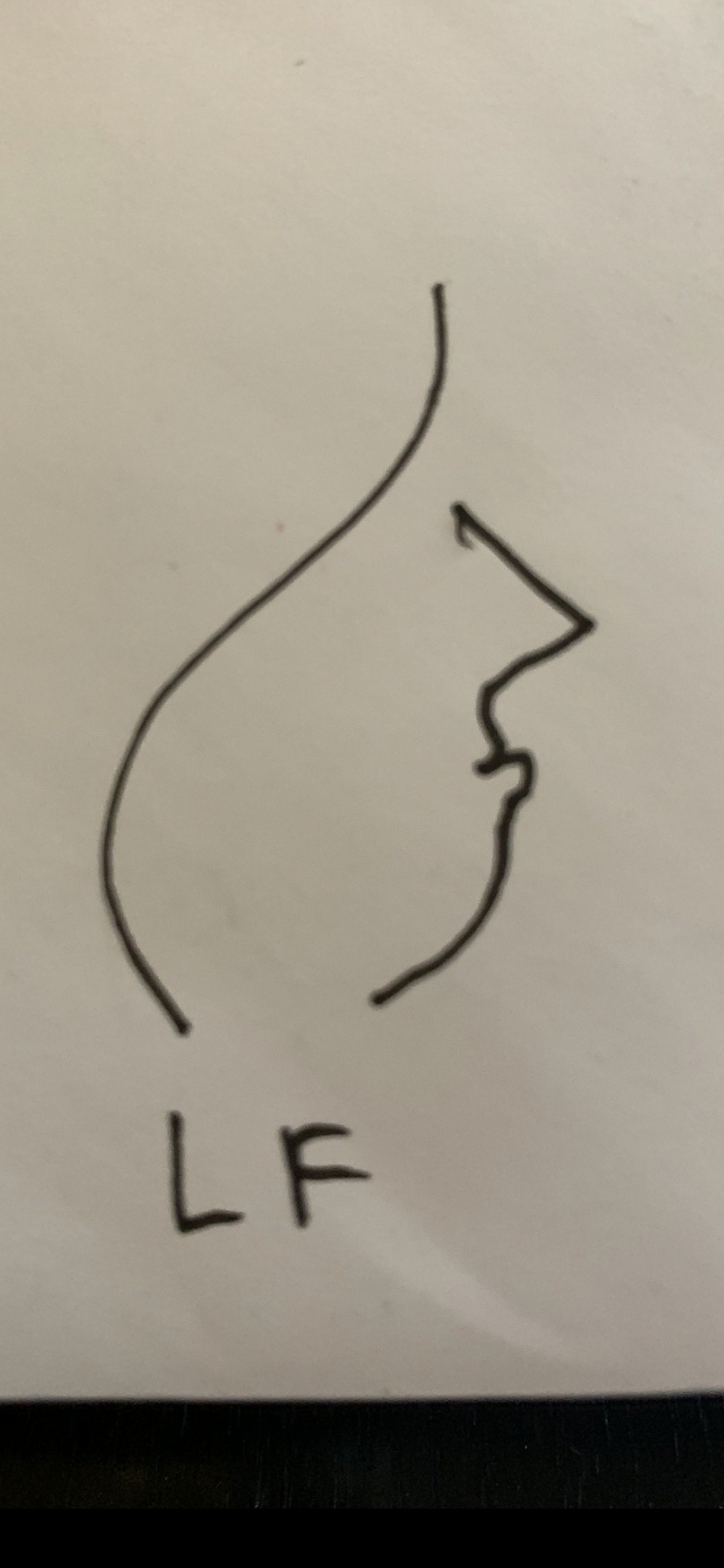A black and white photograph captures a slightly crumpled white piece of paper positioned on a black surface. The black surface is subtly visible at the bottom couple of inches of the paper. The paper features a black felt-tip sketch that starts at the top center, with the pen creating a flowing line that initially curves down and slightly to the left, forming a gentle wave. This line then sweeps into a more pronounced curve before abruptly stopping, resembling the form of a wiggly snake. To the right of this snake-like line, a pyramid-like shape begins a little lower down the page; it curves outward into a protruding lip and possibly a chin, suggesting the features of a face. The overall image brings to mind a juxtaposition between the left side, which appears vase-like, and the right side, which resembles facial features. Below this abstract composition are the handwritten initials "L" for Lima and "F" for Freddie. The paper's surface is not smooth; a faint crease indicates it has been scrunched up previously.